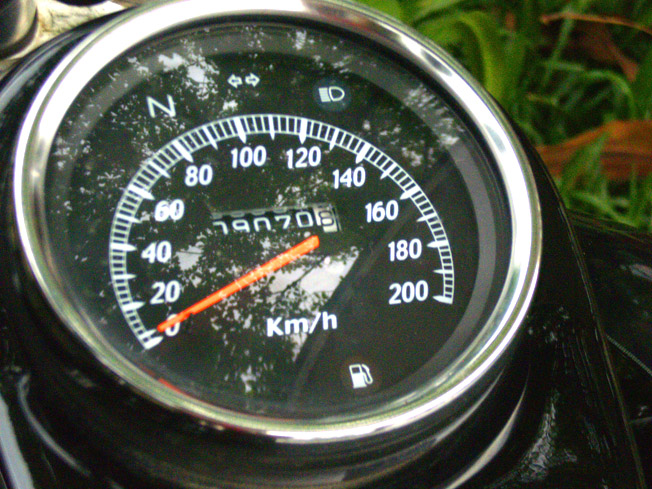This detailed photograph captures the speedometer of a two-wheeled vehicle, likely a motorcycle or scooter, given its positioning and the black leather-like material that appears beneath it. The background of the image features green grass and red leaves, suggesting the vehicle is outdoors, which supports the inference that it is not a car speedometer. 

The speedometer is encased in a circular silver metal border. Within this border, a digital readout is visible, displaying various indicators: neutral, left and right blinkers, and high beam lights. Additionally, a small illuminated circle at the bottom showcases a gas station fill-up icon. The analog gauge ranges from 0 to 200 kilometers per hour, with an orange needle pointing to zero. Notably, the mileage readout in the center of the speedometer displays 90,708 kilometers.